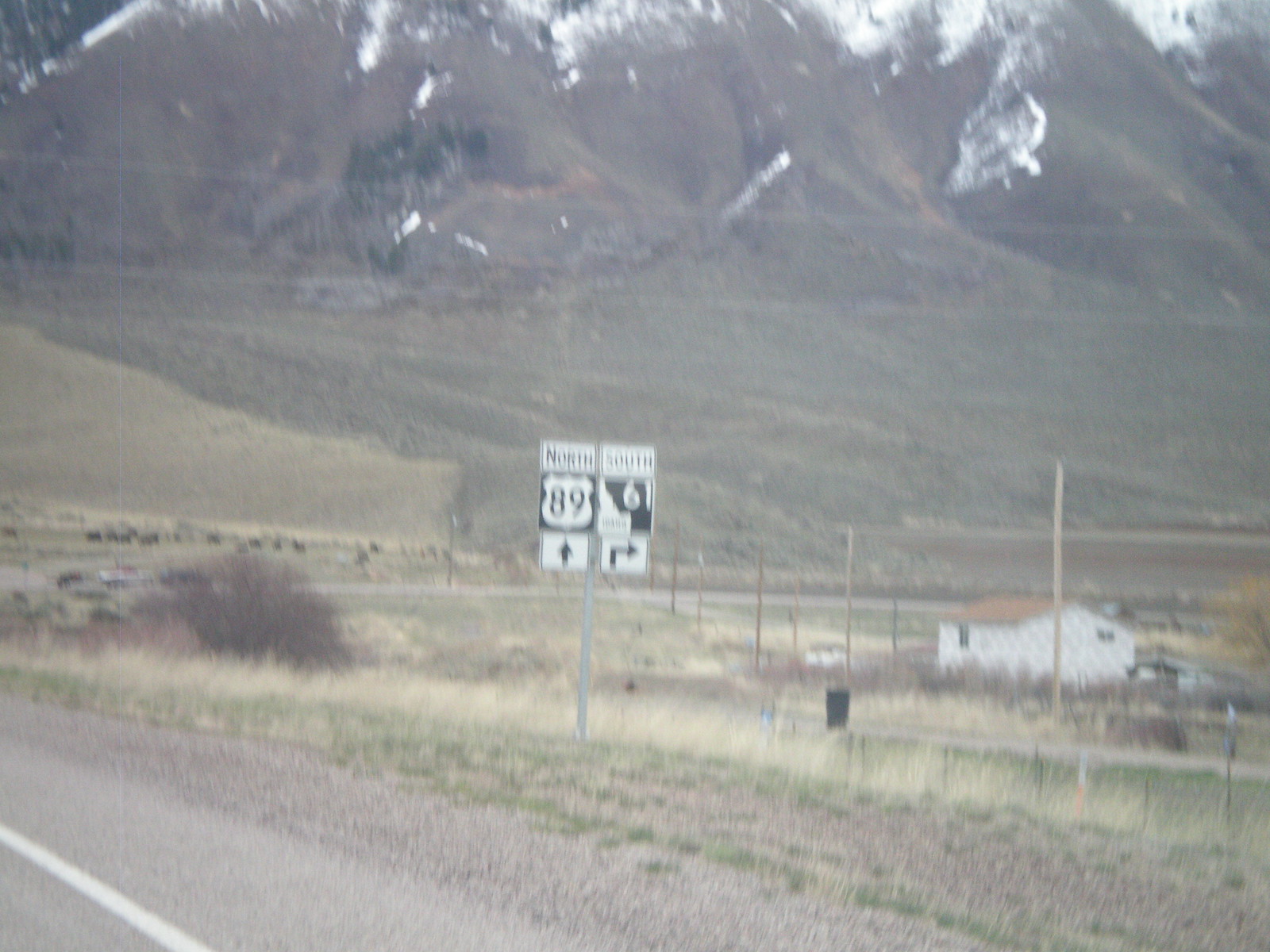A detailed map illustrating a route where North 89 is indicated by an upward-pointing arrow. On the right side, South 61 is denoted with an arrow pointing to the right. At the top of the map, picturesque mountains capped with white snow dominate the scenery. In the bottom right corner, a rustic stone house with a brown roof is visible. On the left side of the image, a solitary brown tree stands prominently. The map appears to depict a highway in Idaho. Additionally, a farmhouse with partial visibility is situated on the right side, adding a quaint rural touch to the landscape.